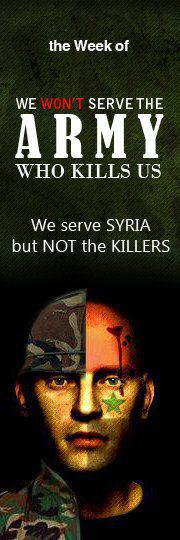This is a detailed poster design. The top features bold white text against a black background, stating: "The Week Of We Won't Serve The Army Who Kills Us. We Serve Syria But Not The Killers." The message emphasizes resistance against oppressive forces while standing in solidarity with Syria.

Below the text, there is a compelling and symbolic image of a man with a divided appearance. The left side of his face is bald, featuring a green star under his eye and a red heart on his forehead that appears to be dripping blood into his eye. His lips are painted red. He wears a black t-shirt on the left side of his body. The right side of his head shows him wearing a camouflage military cap and corresponding army jacket in shades of green, yellow, brown, and black. The stark contrast between the two sides of his appearance underscores the internal conflict and the poignant message of the poster.